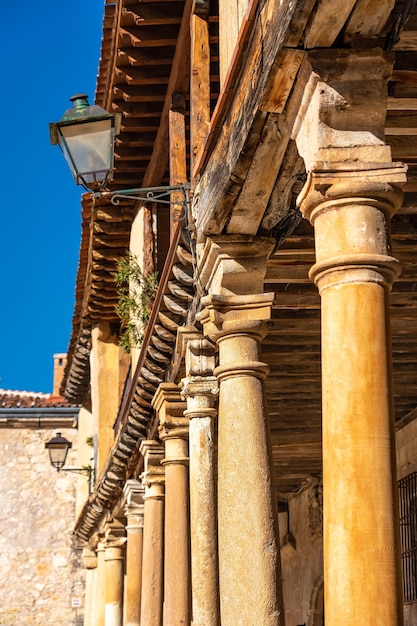This image captures a vertical, rectangular view looking up at a line of ancient stone pillars, which appear weathered with a yellowish, white hue and brown decay, indicating their old age. There are precisely eight columns, each subtly unique, suggesting they may have been installed at different times. These stone pillars support a second story made of distressed wood, characteristic of ancient architectural designs likely dating back to Roman times. Mounted on L-shaped brackets attached to the upper structure, there are antique metal and glass sconces that appear to be from the 1500s. The scene portrays the juxtaposition of the robust stone pillars and the old wooden structure above, creating a harmonious yet historic atmosphere. The sky is visible on the left side of the image, while the right showcases the juxtaposition of the stone pillars with the antiquated wooden or possibly brick building.